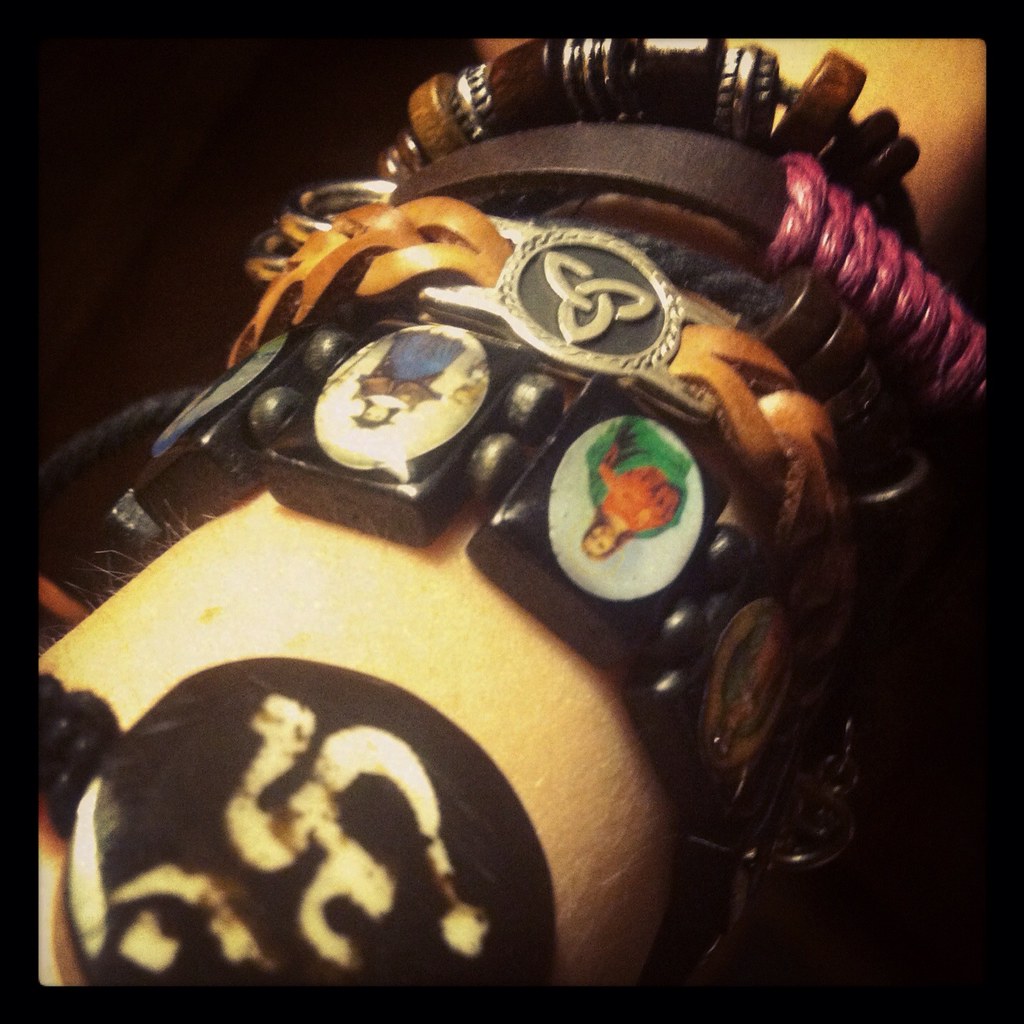In this close-up image against a totally black background, a person's fair-skinned arm adorned with a series of distinctive bracelets is prominently featured. The arm, sprinkled with fine, light hairs, wears a variety of bracelets, each more detailed than the last. Starting from closest to the hand, there is a bracelet adorned with brown wooden ornaments, followed by one made of brown rawhide braided with purple string and featuring a silver emblem. An orange bracelet with a gold clasp rests above, and further up, a striking bracelet displays small black squares interspersed with tiny black beads, each square showing intricate portraits of what seem to be saints and Jesus, depicting an antique style. There is a notable bracelet with an oval-shaped picture of a woman in a green dress with red accents, alongside another portrait, likely dating from the early 1900s. Additionally, there is a leather thong with pink rope detail, and towards the elbow, a blue rope bracelet accented with brown beads. The diverse textures and historical nuances of the bracelets create a rich tapestry of adornment on the arm, captured brilliantly against the dark background.